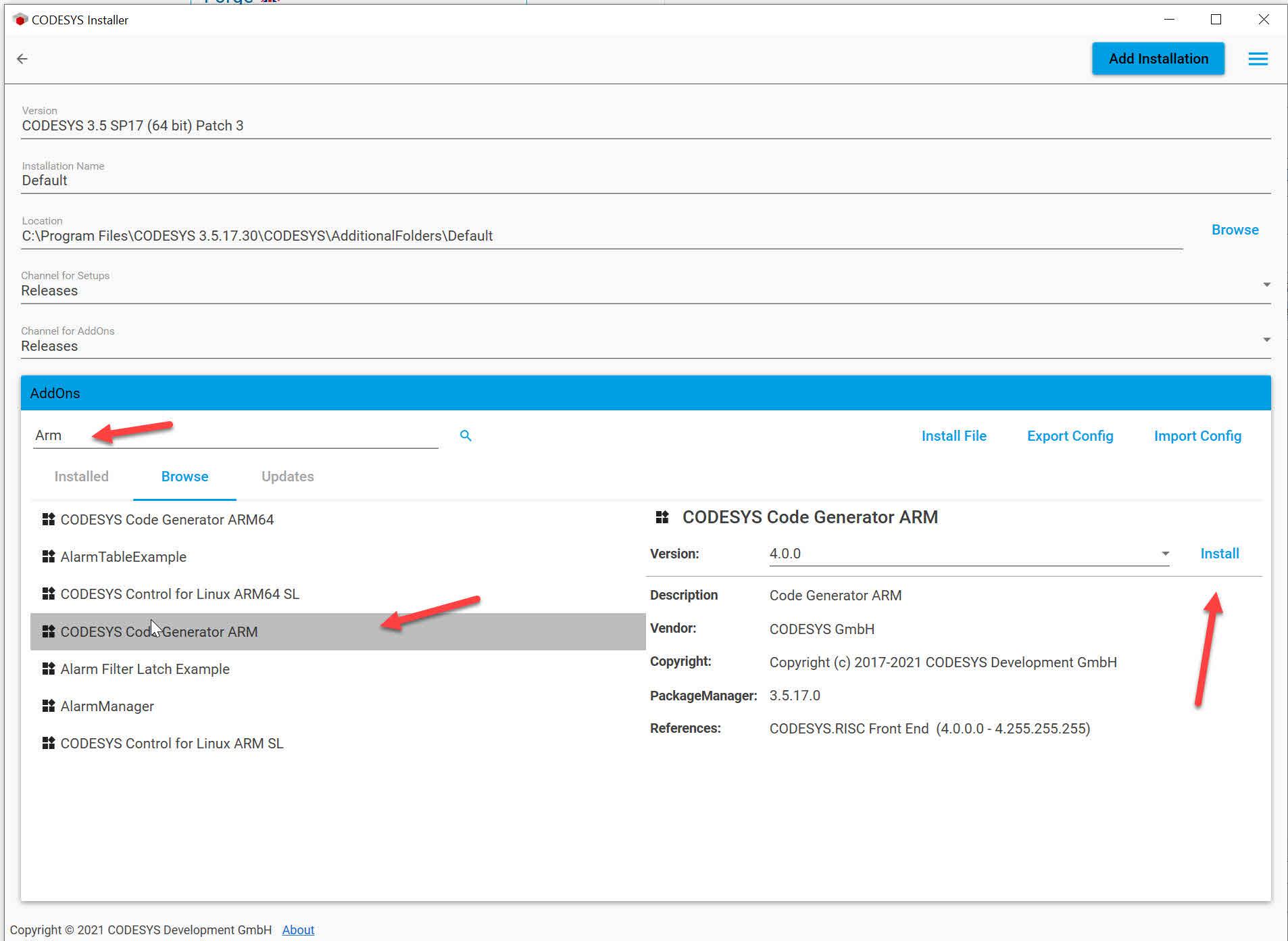The screenshot displays a window titled "Code SYS Installer," featuring a technical interface dedicated to managing software installations. The header indicates the application is the "Code SYS 3.5" version, specifically the SP 17, 64-bit version, patched to version 3. Below the title, fields for "Version Name" and "Default Location" are visible, with the default location showing a file path within the "Program Files" directory.

The interface further comprises sections labeled "Channel for Setup" and "Channel for Add-ons," both set to "Releases." A smaller sub-window titled "Add-ons" is located below these controls. Within this sub-window, the user has searched for the term "ARM," referring to a type of micro-architecture typically used in low-level code operations.

Tabs across the sub-window are labeled "Installed," "Browse," and "Updated on Browse," with a list of add-ons presented therein. A specific add-on, "Code SYS Code Generator ARM," is selected. On the right side, detailed information is shown: the add-on is identified as version 4.0, and it is managed by Package Manager 3.5.17. Notably, there are arrows pointing towards an "Install" button on the right side, highlighting the next step for the user.